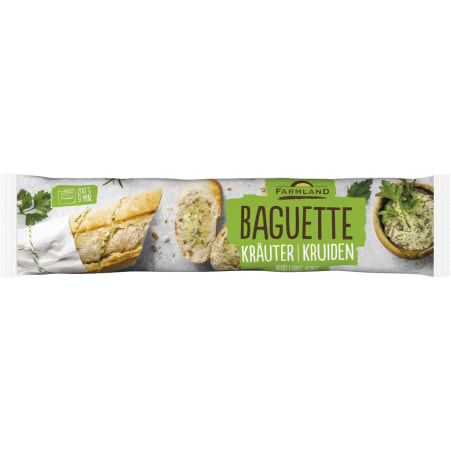The image displays a vertically oriented, thin rectangular package of a frozen baguette, set against a plain white background with occasional touches of white on either side. The packaging itself is predominantly off-white, adorned with images of cut-up baguette slices garnished with garlic, butter, and green garnish. The left half of the package showcases pieces of the baguette facing up, while a whole baguette, sliced down the middle, is prominently featured, appearing to extend out from the packaging. Above the sliced baguette, a small green rectangle likely contains nutritional information.

Central to the design is the branding: the words "Farmland" appear in dark brown text with an underline and a half-sun emblem above it, situated on a green background. Beneath this, "Baguette" is written in capital letters, followed by "Crauter," with an umlaut over the 'a,' in white text. A white dividing line separates this, leading to the word "Kruiden." To the right of these texts is a wooden bowl filled with a dip-like substance, garnished with green herbs. A leaf and a decorative bow with a small plant sticking out add to the rustic, farm-fresh aesthetic of the packaging.